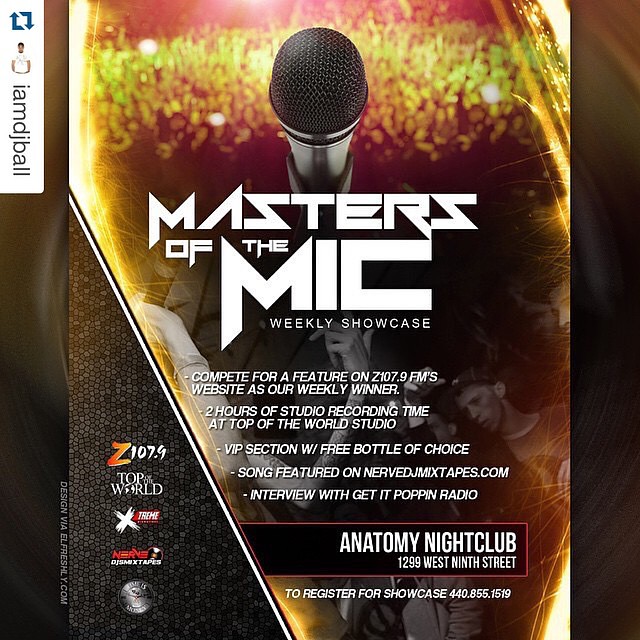This image is a promotional poster for the "Masters of the Mic Weekly Showcase." The background of the poster features a blurred concert audience viewed from the stage, creating an energetic atmosphere. Superimposed in the center is a prominent microphone. The main text, in sharp white letters with angular styling, reads "Masters of the Mic Weekly Showcase." 

Detailed information follows: "Compete for a feature on Z107.9 FM's website as our weekly winner. Two hours of studio recording time at Top of the World Studio. VIP section with free bottle of choice. Song featured on NerveDJMixTapes.com. Interview with Get It Poppin' Radio."

At the bottom, the event location is specified: "Anatomy Nightclub, 1299 West 9th Street." To register for the showcase, the contact number is provided: "440-855-1519."

The poster includes a vertical border on both sides. On the left side, there's an upper-left white vertical rectangle with an image of a man and the text "I am DJ Ball" written vertically. Below this, various sponsor logos are displayed on a gray triangle, including "Z107.9," "Top of the World," "Extreme," and "NerveDJMixTapes.com."

Additionally, in the lower-left corner, it notes, "Design via ELfreshly.com."